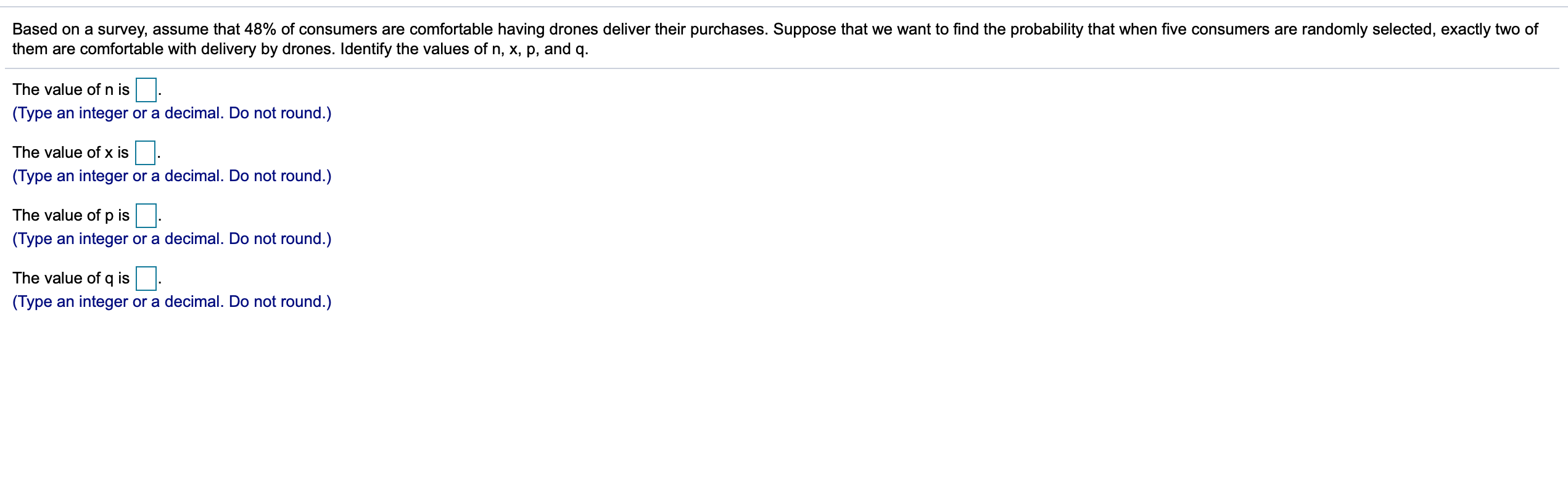The image is a simplistic representation, primarily dominated by a panoramic white background. At the top, black text is positioned between two faint, elongated gray lines, delivering the message: "Based on a survey, assume that 48% of consumers are comfortable having drones deliver their purchases. Suppose that we want to find the probability that when five consumers are randomly selected, exactly two of them are comfortable with delivery by drones. Identify the values of n, x, p, and q."

To the left and towards the bottom, a series of text instructions and blue-highlighted fields appear in sequence:
1. The first line reads: "The value of n," followed by an unmarked blue square. Beneath this, there are blue letters in parentheses instructing: "(type an integer or a decimal, do not round)."
2. The second line specifies: "The value of x," accompanied by another blue line box with a white interior, and similar instructions in parentheses below it.
3. The third line states: "The value of p," once again with the same blue box and white interior, and identical parentheses instructions underneath.
4. The fourth and final line indicates: "The value of q," featuring another blue line square with a white interior, with the same words in parentheses underneath it.

Overall, the setup resembles a problem likely derived from an algebra or math quiz, focusing on probability calculations involving consumer comfort levels with drone-based deliveries.